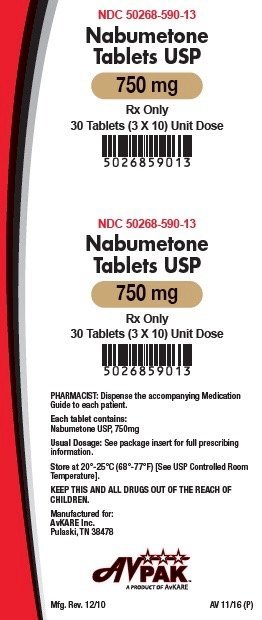This image features a detailed label for a prescription medication, specifically Nabumetone tablets. The overall design is clean and clinical, primarily utilizing a white background complemented by a curved stripe on the left side in shades of red, black, and gray. 

At the top of the label, large black text states:
"NABUMETONE Tablets, USP, 750 mg, RX Only, 30 Tablets (3 x 10 Unit Dose)"
Adjacent to this is a barcode numbered "5026859013".

Reiterating this information, the label again lists:
"NABUMETONE Tablets, USP, 750 mg, RX Only, 30 Tablets".

Further down, a section intended for pharmacists highlights:
"Dispense the accompanying Medication Guide to each patient. Each tablet contains NABUMETONE USP 750 mg. Usual Dosage: See package insert for full prescribing information. Store at 20 to 25 degrees Celsius (68 degrees to 77 degrees Fahrenheit), USP controlled room temperature. Keep this and all drugs out of the reach of children."

The manufacturer and product information specify:
"Manufactured for AAV Care Inc., Pulaski, TN 38478. AAV Pack."

At the bottom, there is a logo and branding text:
"AAV Pack, a product of AAV Care," followed by identifiers "AAV 1116" and "MFG REV 1210".

This comprehensive label ensures all vital prescribing guidelines, storage instructions, and manufacturer details are clearly communicated.